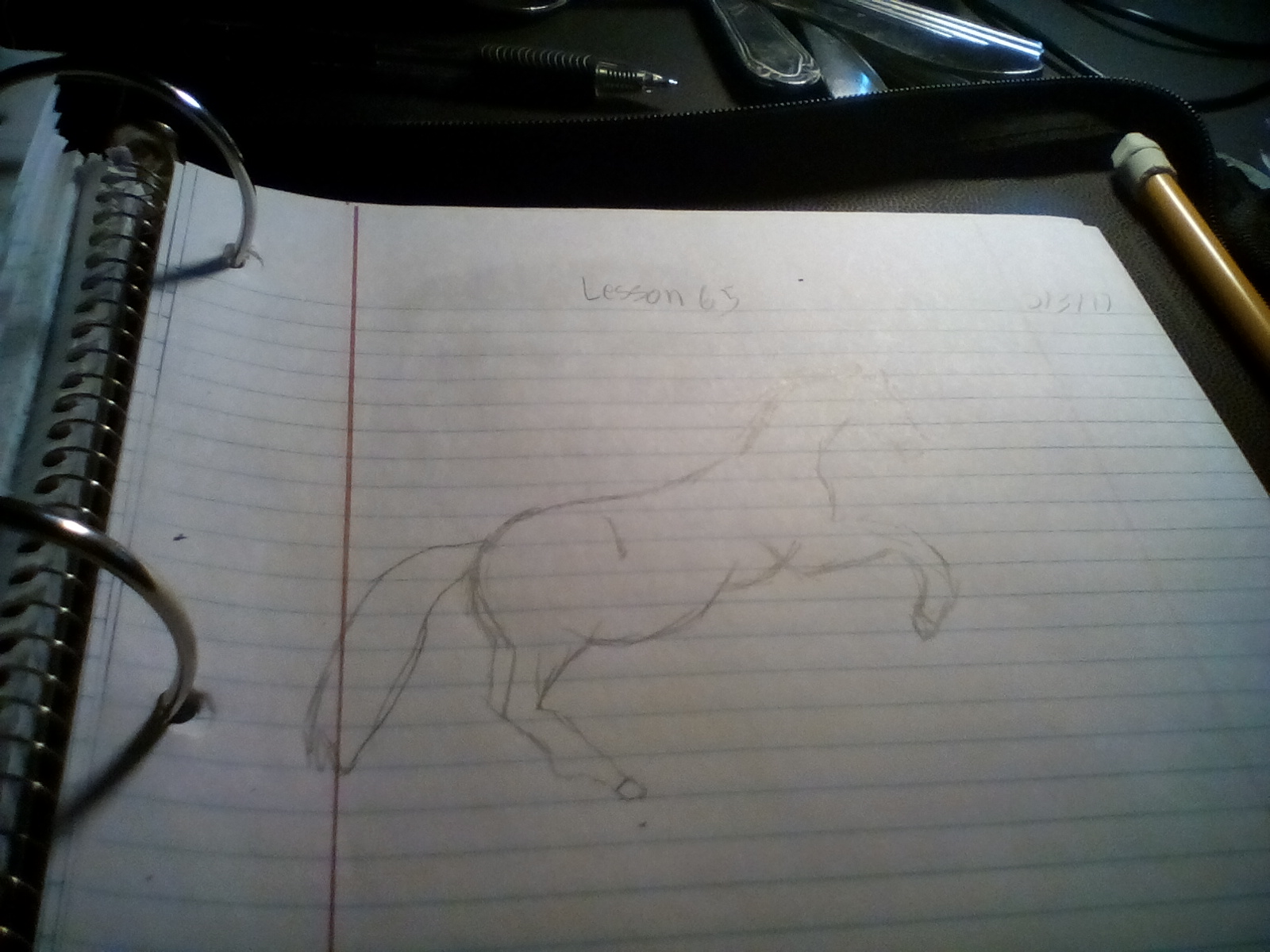This photograph captures a detailed desktop scene. Dominating the image is an open three-ring binder with a fabric cover, resting on what appears to be a black desktop background. The binder holds a piece of lined paper, hole-punched and with a red vertical margin line on the left. At the top of this paper, it reads "Lesson 65." The primary focus of the paper is a pencil drawing of a horse rearing up on its hind legs, facing right. The horse's front legs are raised, suggesting motion, and it has a long, flowing tail.

In the upper center portion of the photo, there's an ink pen. Above the binder, some silverware can be seen, and to the right, a copper pipe with a metal end piece is visible. The image gives a sense of cluttered creativity and schoolwork, combining everyday objects with an artistic sketch.